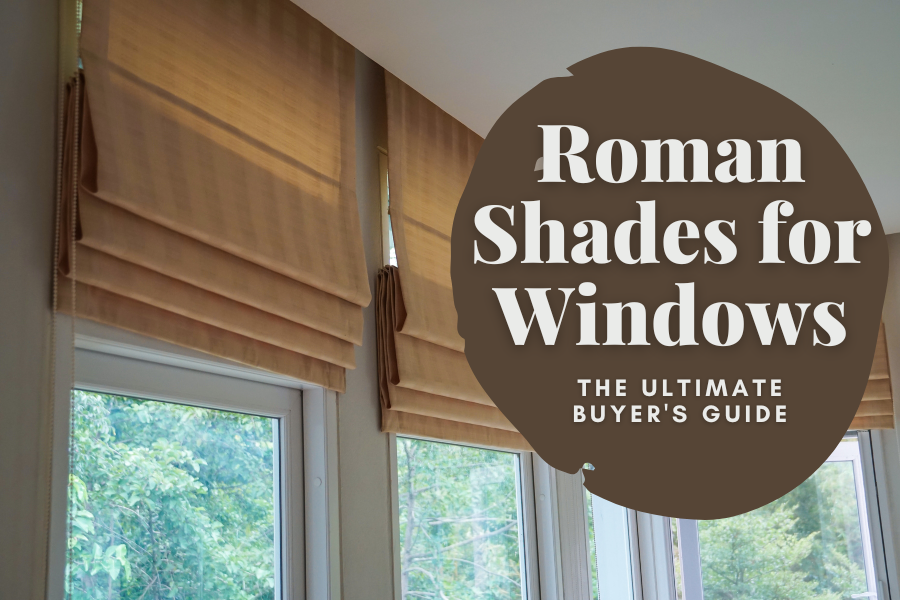The image serves as an informational cover for a buyer's guide on Roman shades for windows. Dominating the visual is the corner of a house featuring three tall windows with white trim, each adorned with folded, dark tan Roman shades. These shades are pulled up, showcasing their neatly folded design that resembles overlapping fabric rather than an accordion style. In the foreground, there's a prominent brown circle that mimics the look of a tree trunk cross-section. This circle contains white text stating "Roman Shades for Windows" and just below, it reads "The Ultimate Buyer's Guide." Outside the windows, lush green trees are visible, suggesting a forest or backyard scene illuminated by daytime sunlight.